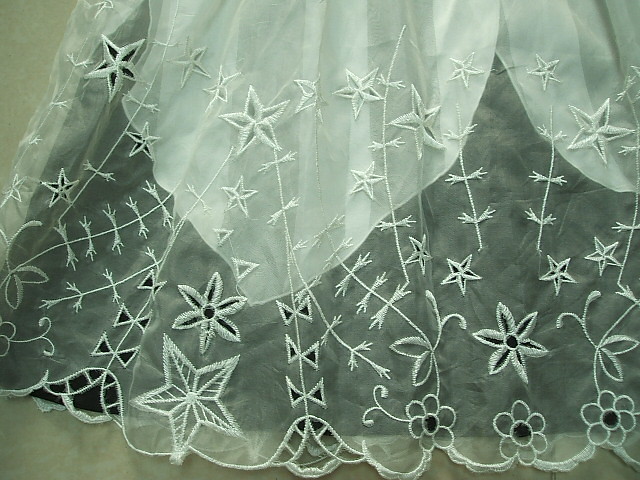This square image prominently features the bottom part of a lacy wedding dress, positioned centrally against a background likely consisting of gray and greenish tile that appears to be indoors. The lace fabric, sheer and delicate, showcases an intricate pattern of flower stems that culminate in stars, with additional scattered stars boasting various designs. Underneath this ornate lace layer is a darker-colored fabric, adding depth and contrast, and another solid white layer visible near the knee area. The photograph, devoid of any text or other objects, captures a palette of white, off-white, black, and gray, creating an elegant and detailed depiction of the dress’s elaborate design.